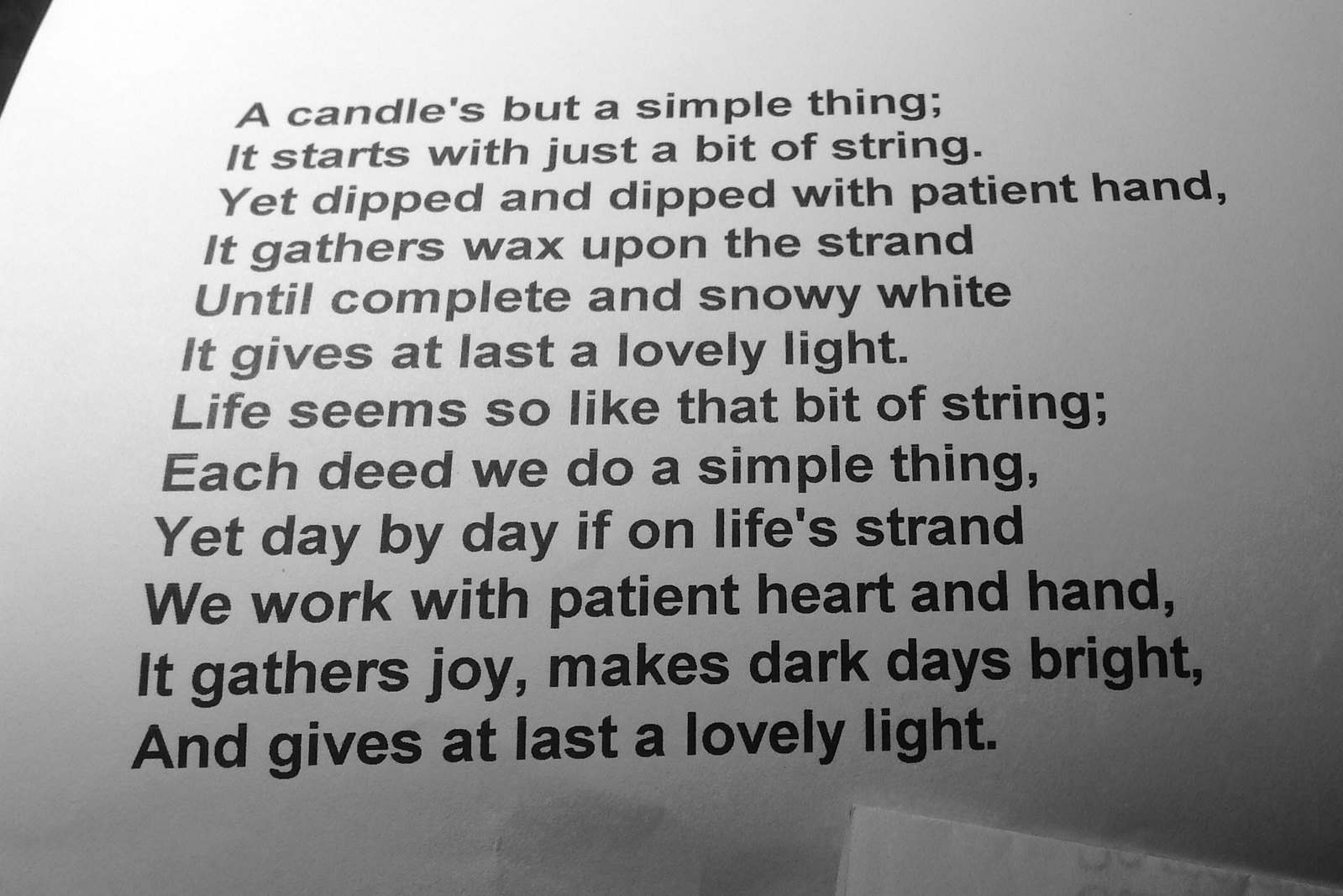This image features a poem printed in black text on a sheet of white paper, which appears slightly wrinkled and is positioned at an angle, creating a glare in the top left corner. The poem reads: "A candle's but a simple thing. It starts with just a bit of string. Yet dipped and dipped with patient hand, it gathers wax upon the strand. Until complete and snowy white, it gives at last a lovely light. Life seems so like that bit of string. Each deed we do a simple thing. Yet day by day, if on life's strand, we work with patient heart and hand. It gathers joy, makes dark days bright, and gives at last a lovely light." In the very top left corner, part of another object is visible behind the paper, appearing black. In the bottom right corner, another piece of paper, likely folded, rests on top of the main sheet. The poem, set in a basic font, draws a parallel between the process of making a candle and life's incremental joys and brightness derived from persistent efforts.